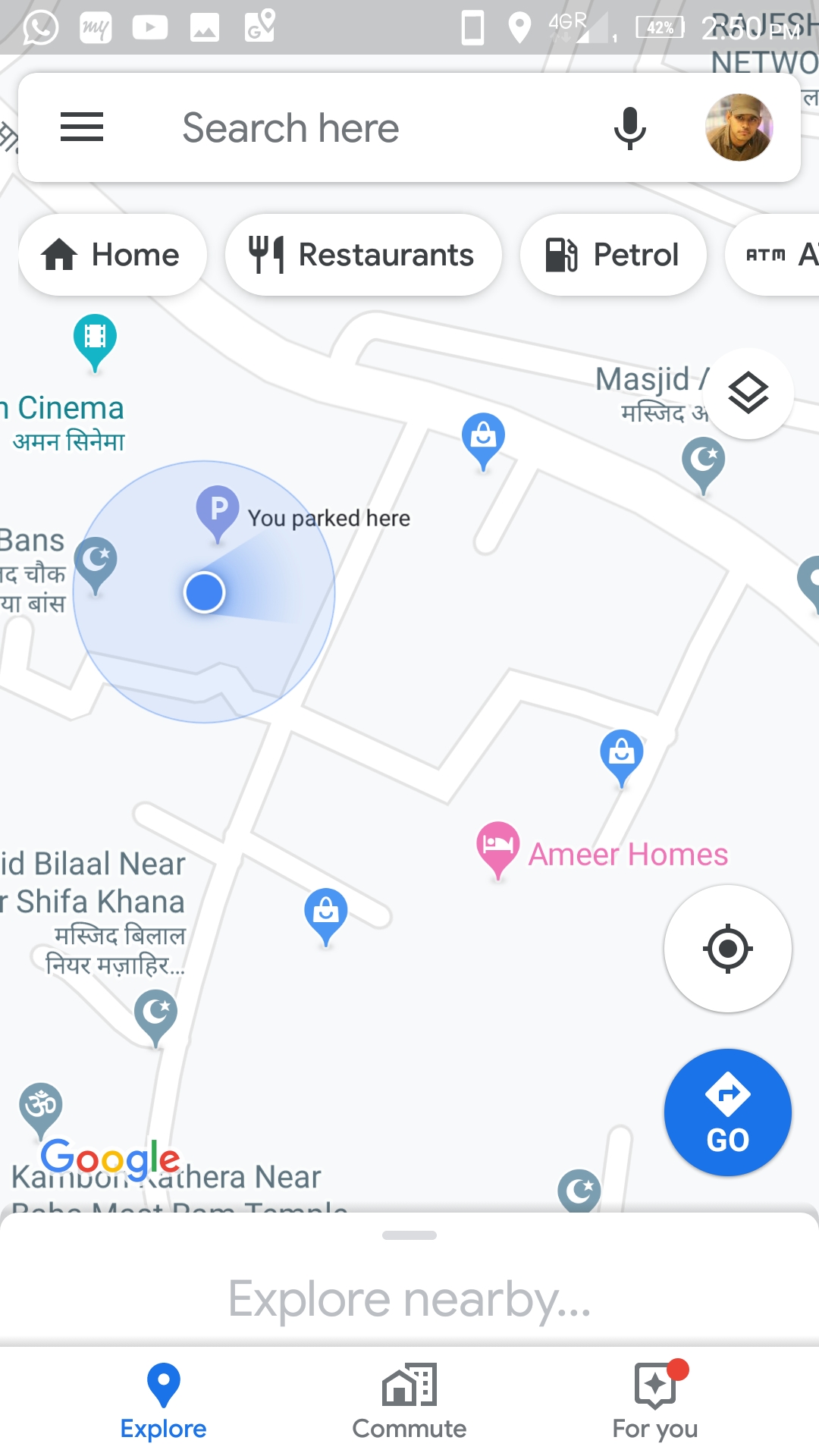This screenshot depicts a detailed map of a neighborhood, highlighting several key features and locations. The focal point of the map is Amir Homes, marked prominently in pink. Various roadways crisscross the area, with significant markers to aid navigation. On the left-hand side, a blue circle with a lighter, larger circle around it indicates the user's current parked location, labeled with a "P". In the same vicinity, a marker with a half-moon and star symbolizes the location of a cinema.

The map includes both English text and another language, possibly reflecting a region such as Afghanistan. The top section of the screenshot is grayed out with several icons, including a chat bubble, phone, directional arrow, marker, Wi-Fi, battery usage, and the time displayed as 2:50 p.m.

Below these icons, there is a search bar with a microphone icon and a rounded profile picture next to it. On the left side of the search bar, three horizontal lines serve as a menu icon. Beneath the search bar, four category buttons are partially visible: home, restaurants, patrol, and another cut-off category.

The map itself is detailed, featuring multiple roads and markers. In the lower-left corner, the Google logo appears in its traditional blue, red, yellow, and green colors, occupying minimal space. Adjacent to it, on the right-hand side, is a blue circle with the word "Go" and a directional arrow.

Below these elements, "Explore nearby" is written in gray, suggesting it as a search prompt. Further down, there are three tabs: "Explore," highlighted with a blue marker icon; "Commute," in gray with a building icon; and "For you," displaying a chat bubble within a square, a four-pointed star, and a red notification dot in the upper right corner of the icon.